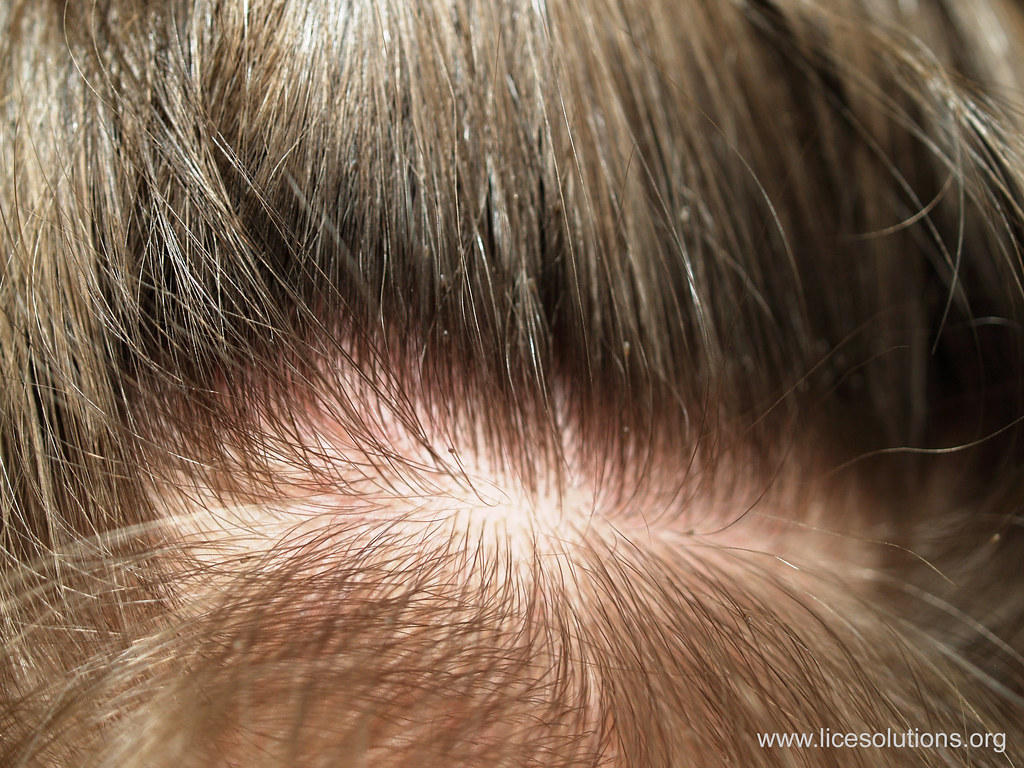This is an extremely close-up, high-quality, landscape-oriented photograph focused on a person’s scalp, revealing a slightly pink Caucasian skin tone. The hair, which is mostly dark brown with a few minor gray strands, is parted down the center, exposing the scalp in several places, suggesting the hair is fine in texture, thin, or possibly thinning. The part in the hair clearly displays the white scalp of the individual, and interspersed within the hair are tiny black lice and their eggs, resembling small black seeds. Some of these lice and eggs are visible near the parted area. The image is credited in the lower right corner to www.lyssolutions.org.